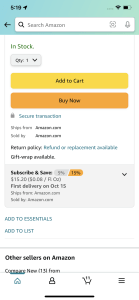A detailed caption for the described image could be:

“A user’s smartphone displaying an Amazon product page at 5:19 PM, with a nearly full battery indicator. At the top, there is a light blue banner featuring a search bar with the prompt ‘search Amazon’. Below, green text indicates 'in stock,' followed by ‘quantity: one’. Options to ‘Add to Cart’ or 'Buy Now' are prominently displayed, along with return policy information. Below, light blue text states ‘refund or replacement available’ and ‘gift wrap available’. A light gray box below provides a ‘Subscribe and Save’ option, though the text within is blurry. Additional options include 'Add to Essentials' and 'Add to List' in light blue text. Information about other sellers on Amazon is partially visible but cut off.”